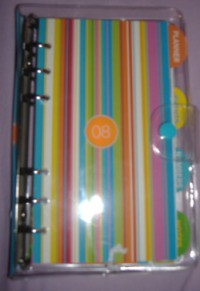This photograph, taken in portrait orientation against a mauve or pink background, captures an image of a vertically-striped notebook with multiple colors such as red, white, blue, yellow, orange, green, and purple. The reflective white mark on the notebook indicates the photo was taken with a cell phone flash. The notebook, slightly out of focus, is encased in a protective plastic cover with a snap closure, and features a six-ring binding system, with three rings at the top and three at the bottom. Centered on the striped cover is a prominent orange circle bearing the number 08, outlined with a white rim. Along the right edge of the notebook, visible through the plastic cover, are colorful tabs in orange, yellow, blue, and green, which likely separate different sections within the notebook. The silver rings and the popper closure further add to the notebook's functional design.